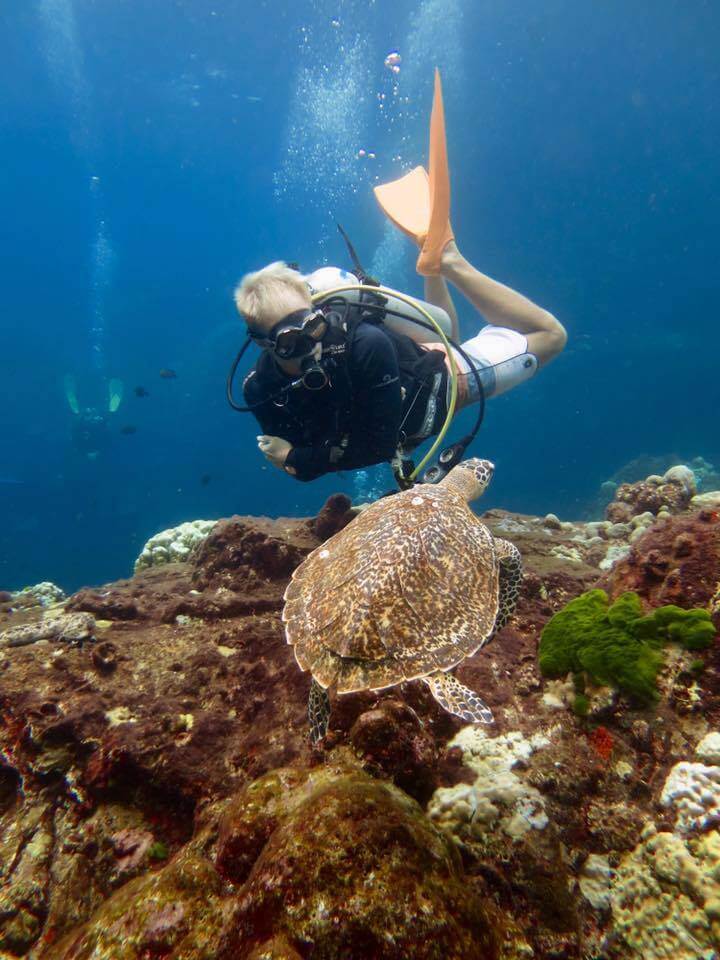This underwater photograph captures a scene teeming with marine life and human activity. At its center, a male scuba diver gazes at a large, mottled tan and gray sea turtle with black eyes, which is swimming gracefully above a mound of brown and gray coral adorned with green moss. The diver, identified by his light blonde hair and slightly balding head, is equipped with a silver metal oxygen canister on his back, a breathing apparatus in his mouth, and dark goggles over his eyes. He is dressed in a dark blue long-sleeved top and white, blue, and orange striped surfing shorts, and his feet are adorned with orange flippers. Behind him, the azure expanse of the ocean is dotted with rising white bubbles, indicating the presence of two additional divers visible in the distant background. The entire scene is bathed in the serene blue light of the underwater world, highlighting the interactions between human and marine life.